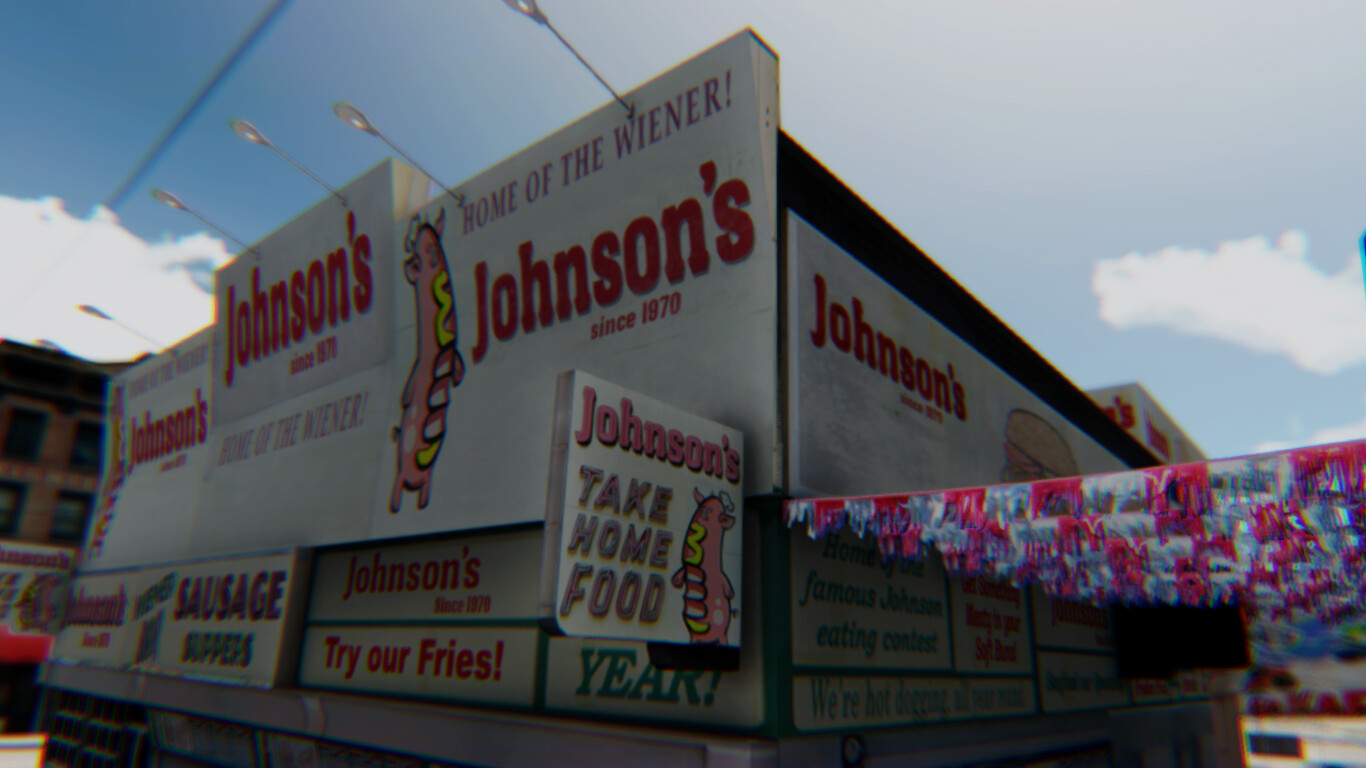This photograph captures a slightly blurry, horizontally aligned rectangular image of Johnson's, an iconic hot dog stand known for its vibrant and nostalgic atmosphere. The top of the image displays a mostly clear blue sky adorned with some puffy white clouds on either side. The scene below reveals a bustling event at the stand, adorned with a plethora of colorful signs and banners. 

At the forefront is a prominent cardboard wall with several darts sticking out from its left side, suggesting some playful activity or contest. The wall prominently features the name "Johnson's" in bold red letters, repeated three times, alongside the slogan "Home of the Wiener since 1970." Accompanying these text elements is an animated depiction of a hot dog with mustard. Below, another sign reads "Johnson's Take-Home Food" along with a similar image of a hot dog. 

A variety of smaller signs cascade beneath, offering tasty enticements such as "Try our Fries," "Sausage Peppers," and mentions of their "Famous Eating Contest." To enhance the festive atmosphere, red, white, and blue banners with fringe hang from the middle, extending to the right side, reminiscent of decorative streamers often found at car dealerships. 

The overall depiction suggests a lively, time-honored eatery that has been delighting customers with its nostalgic charm and delicious offerings since 1970.